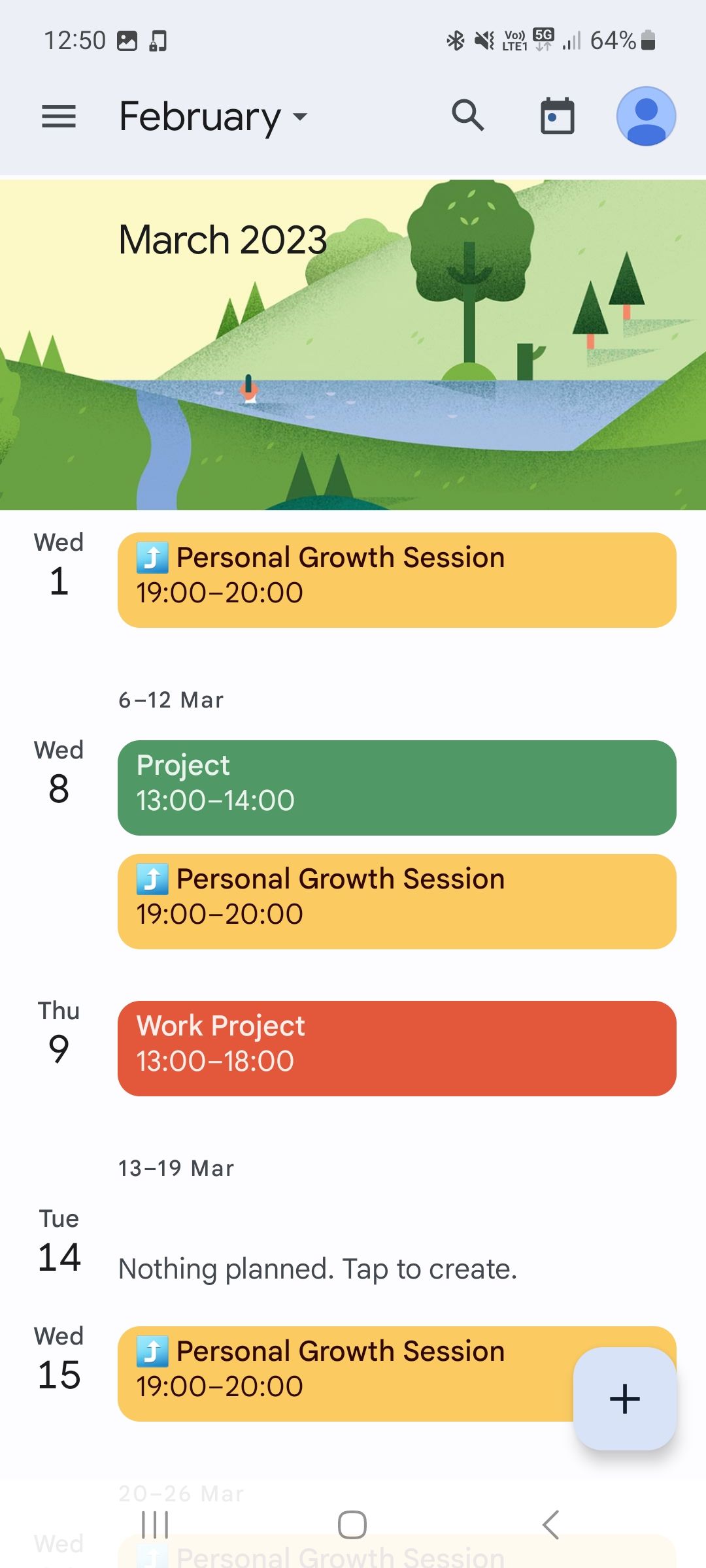The screenshot displays a Google Calendar app on a mobile phone with a current battery level of 64%, taken at 12:50 PM. The calendar is set to the month of March 2023, featuring a color-coded schedule. Highlighted events include a "Personal Growth Session" on Wednesday, March 1st, marked in yellow, a green-labeled "Project" and another yellow "Personal Growth Session" on March 8th, a red-tagged "Work Project" on March 9th, and a final yellow "Personal Growth Session" on March 15th. Despite its organization by color, the calendar doesn’t appear overly busy, showcasing a balanced approach to planning and productivity.